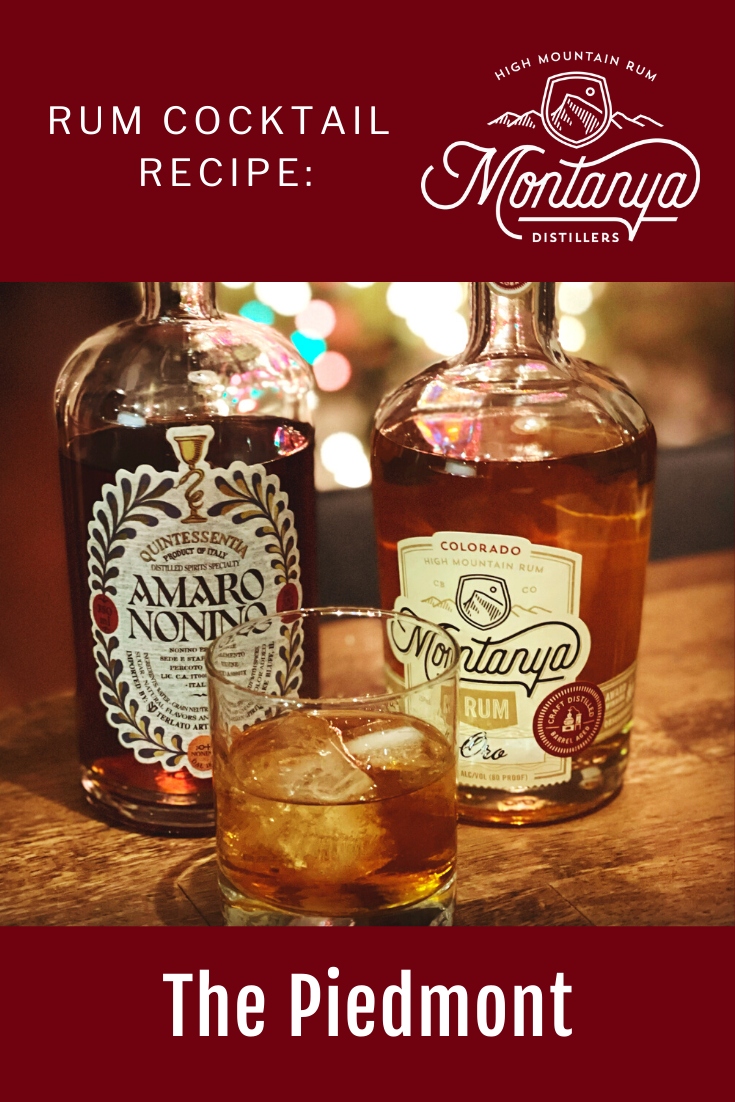The image is a magazine advertisement for Montagna Distillers featuring their rum products. The advertisement is framed with top and bottom banner strips in a rich burgundy color with white lettering. The top strip reads "Rum Cocktail Recipe" followed by the Montagna Distillers logo in cursive. Prominently in the center are two bottles of alcoholic beverages: on the left is a tall, clear bottle with dark black liquid labeled "Amaro Nonino," adorned with a green peace leaf and a trophy logo, and on the right is a slightly thicker bottle with amber liquid labeled "Montagna Rum," also marked with a mountain logo at the top. Between the bottles, in the foreground, stands a glass, half-filled with amber liquid and containing two ice cubes. All of these items are situated on a wooden table. The bottom strip of the ad features the text "The Piedmont" in white lettering.